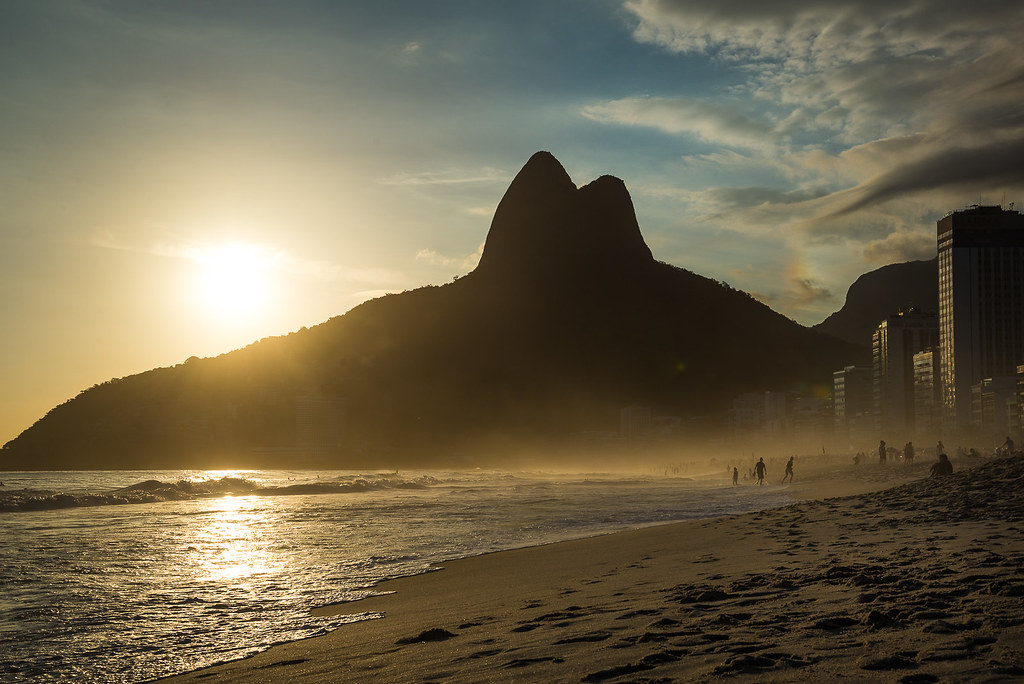In this image, a striking, double-peaked mountain dominates the background, silhouetted against a sky transitioning from blue to the left to slightly cloudy on the right. The sun is low on the horizon, either setting or rising, casting a dramatic yellow glow that reflects off the ocean water, creating high contrast and obscuring much of the mountain's details. Below the mountain, a lively beach scene unfolds, where people frolic and play in the waves. Along the right side of the image, tall buildings, likely part of a beach resort with hotels or condos, line the shore. The beach itself curves gently, with the sand extending into the scene. The overall color palette is dominated by the bright yellow sun, muted blue of the sky, and earthy browns of the beach, underlined by the silhouetted forms of the mountain and buildings.